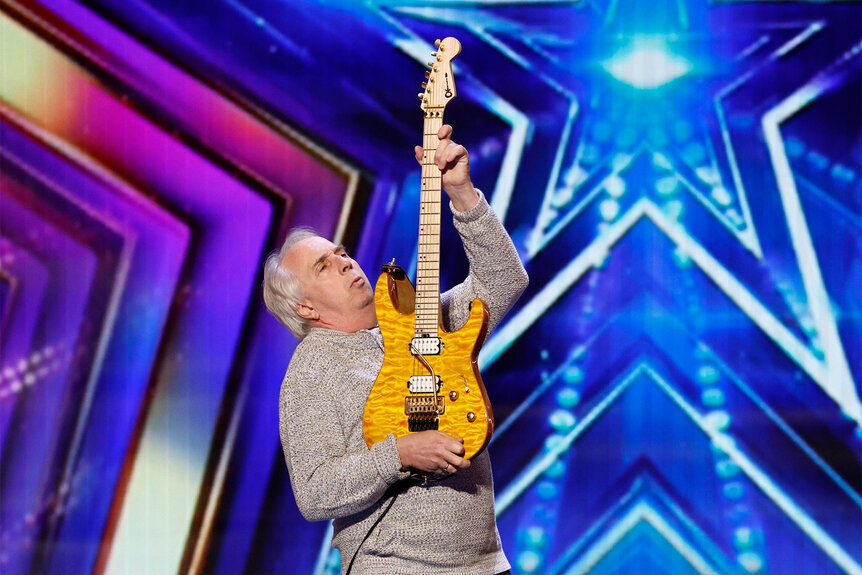An older man, likely in his late 60s, is depicted holding a shiny, golden-yellow electric guitar upright as if he is about to play or pausing mid-song. He is wearing a gray sweater and black pants, with a noticeable ponch and receding, mostly gray hair but dark eyebrows. His eyes are closed, and his head is tilted back, giving his face a stern, expressionless look. His fingers are positioned on the frets while his thumb dampens a string, indicating he knows his guitar techniques. Behind him is a dramatic, rock-themed background featuring ascending star patterns that emit a vibrant blue-cyan light. To the left of these stars, there's a blend of purples, pinks, and golds, forming an intricate scene that evokes the high-energy feel of a talent show like America's Got Talent or American Idol.